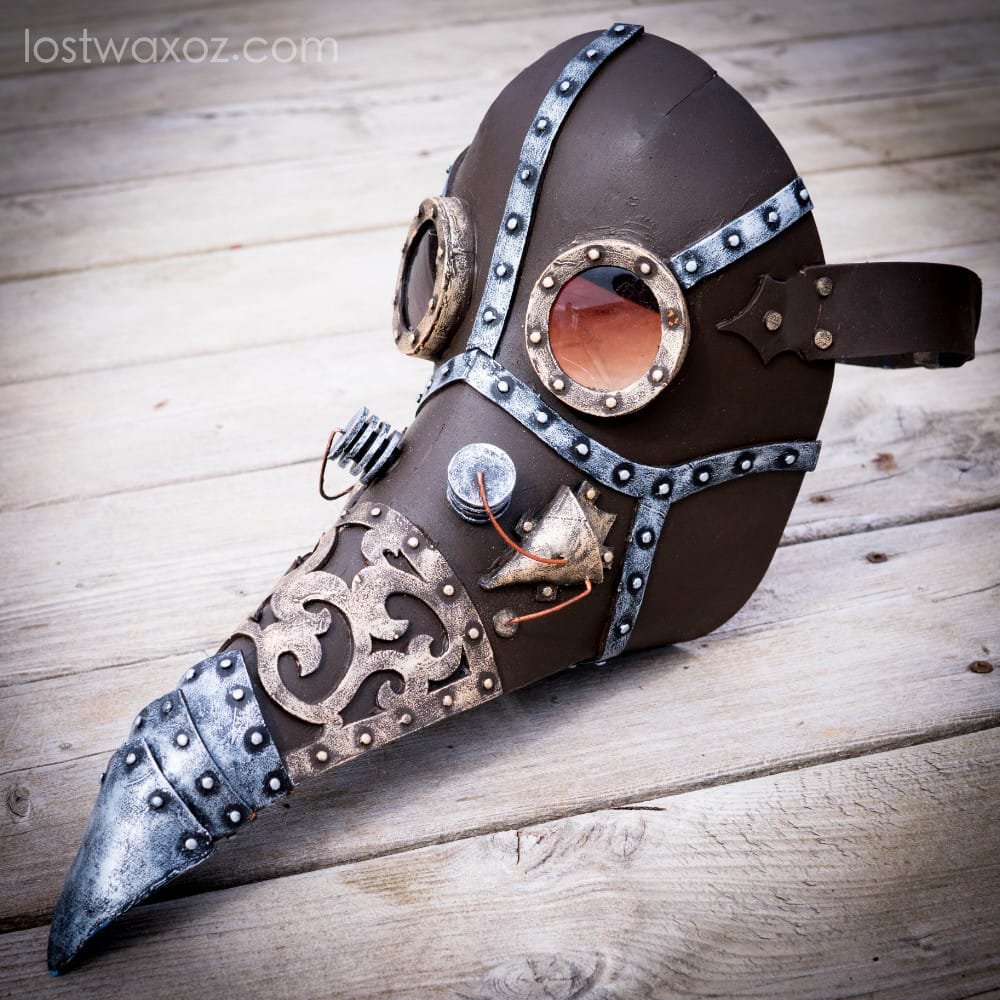This image is a color photograph in portrait orientation featuring a detailed steampunk-style plague doctor's mask. The mask, positioned centrally with its elongated beak pointing towards the bottom left corner, is made of dark brown leather embellished with intricate fretwork of gray steel bands that traverse the forehead, eyes, nose, and cheeks. The eyes have large round openings covered with tinted brown glass, and the nose area, resembling an elephant's trunk, is adorned with multiple steel plates secured with grommets and detailed scrollwork in gold metal. Attached to the top of the beak are two silver cylinders with wires, adding to the mask's steampunk aesthetic. A brown strap is visible, suggesting it's wearable. The mask rests on a light beige, unfinished wooden surface. In the upper left corner of the photograph, a white-screened text reads “LostWaxOz.com”. This highly detailed image combines elements of photographic realism with representationalism, effectively capturing the unique craftsmanship and intricate design of the steampunk mask.